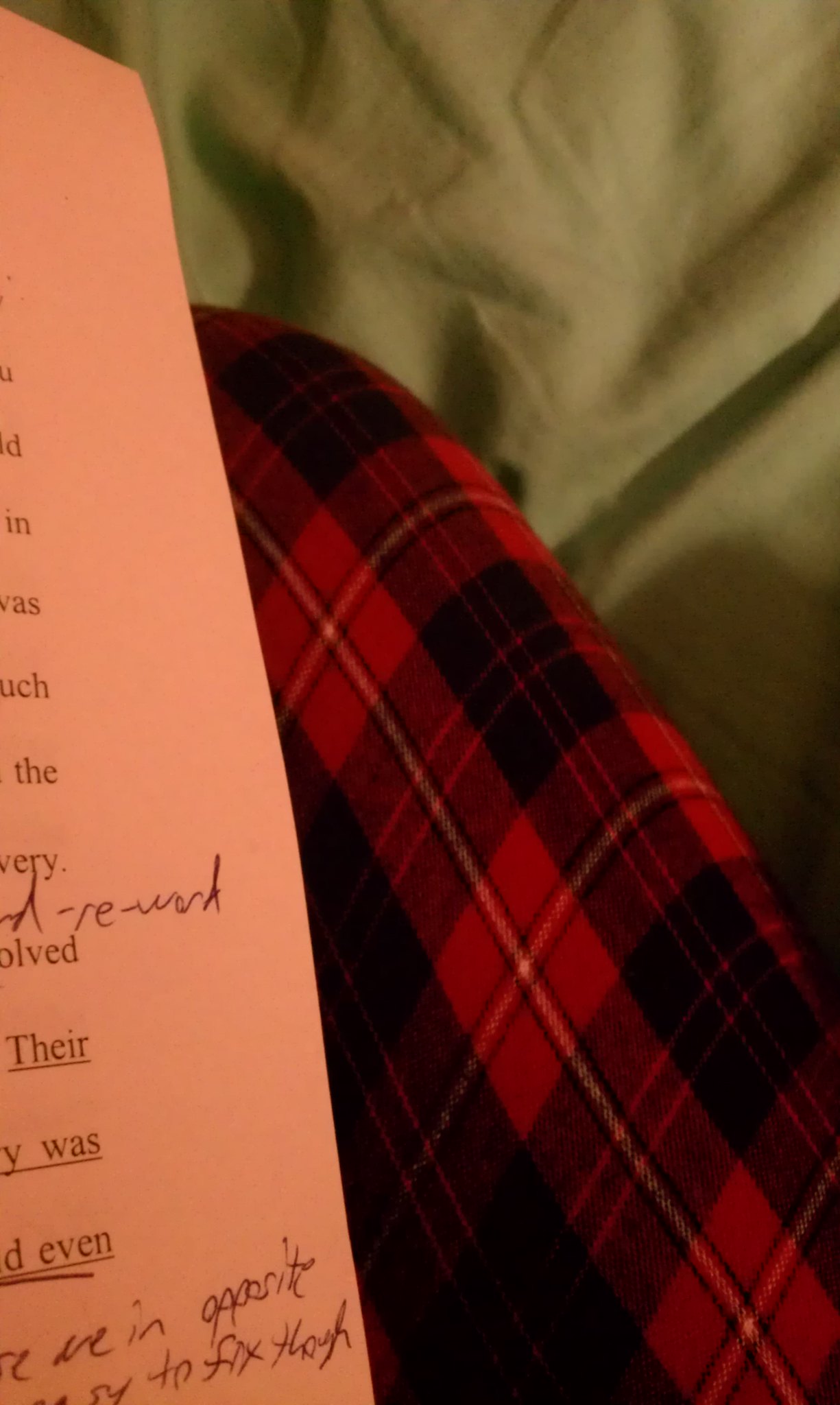The image shows a diagonal view of a chair draped with a red and black plaid cloth, likely the arm or leg of a flannel shirt. Beyond the cloth, the background appears as a light tan or greenish wrinkled sheet, not neatly folded. On the left side of the image, there's an orange piece of paper with both typed and handwritten text. The text on the paper is partially visible, with the words "their," "was," "even," "dash," "re," "wind," and phrases like "we in opposite" and "to fix, though," some written in cursive. The scene suggests someone might be reviewing corrections on the paper, creating a calm, introspective atmosphere.